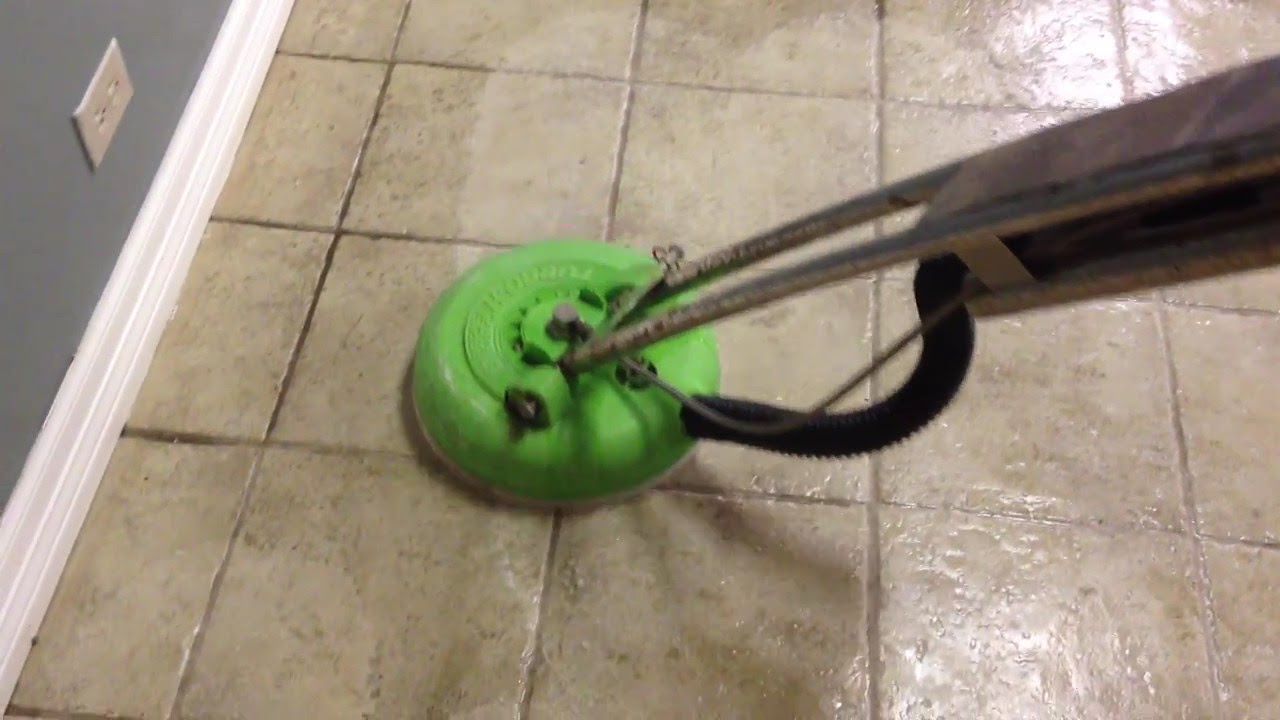The image depicts a man indoors operating an industrial floor cleaning machine with a circular, lime green scrubbing component. The cleaning machine, appearing aged with rusted metal parts, is attached to two metal bars and features a black hose extending from the bottom part of the machine. The man is meticulously scrubbing a tile floor, which is white with a brown speckled design. Notable dirt imprints are visible on the areas yet to be cleaned, highlighting the effectiveness of the machine as it leaves the tiles significantly whiter and cleaner. The setting includes a blue-gray painted wall with a white trim at the bottom, an electrical outlet with a white cover positioned horizontally, and a light switch. The wall and floor meet at a diagonal in the left corner of the image, showcasing the clear contrast between the cleaned and uncleaned sections of the floor.